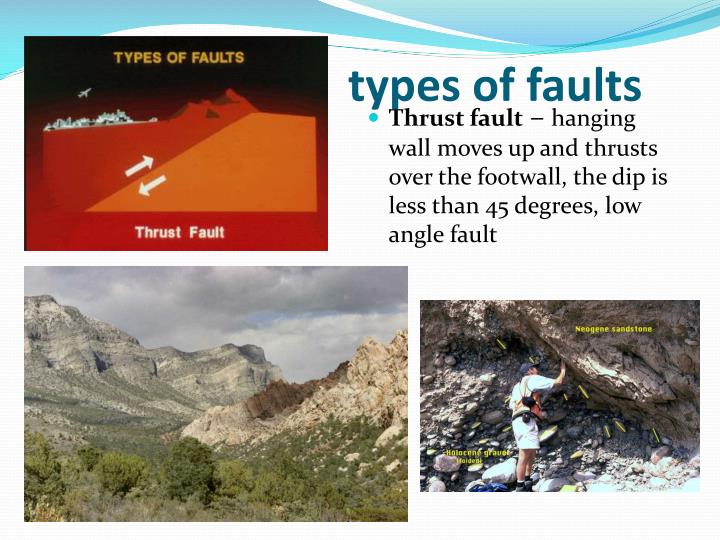This detailed image appears to be a PowerPoint slide or educational poster explaining "Types of Faults." The slide is horizontally aligned and features a clean white background with several prominently placed elements. 

At the top, there are swirled blue and white lines along with a teal title in lowercase letters that reads "types of faults." Beneath the title, a light blue circular bullet point introduces the specific fault type, "thrust fault," in bold black text. The accompanying description explains: "Hanging wall moves up and thrusts over the foot wall. The dip is less than 45 degrees, a low-angle fault."

The image contains three inset pictures. In the upper left corner is a digitally created graphic featuring two fault lines running into each other, highlighted with black, red, and orange colors. White arrows indicate the direction of the fault movement, and this illustration is labeled "thrust fault."

The lower left corner showcases an aerial view of a natural landscape with trees, mountains, and a clear sky.

The lower right corner displays a photograph of a man standing at a cliff or rock formation, identified with signage reading “Neogene Sandstone.” The man, wearing a cap, shirt, shorts, and hiking boots, has a camera slung over his shoulder and is shown with one arm raised, possibly touching or examining the rock face.

In summary, this image effectively combines textual information and visual aids to explain the concept of thrust faults in geology.